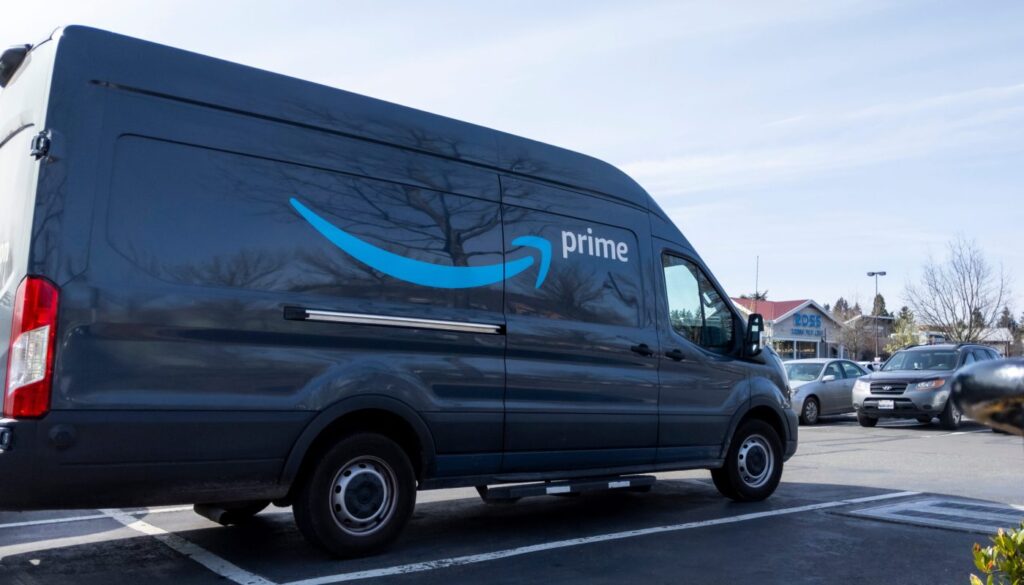The image depicts a webpage screenshot focusing on a black panel van prominently featuring the Amazon Prime grin-with-arrow logo. The van appears to be a Mercedes-Benz, identified by its distinctive design. It is parked in a crowded lot surrounded by various stores. In the background, a Ross Dress for Less store with a red roof is visible. The weather appears to be overcast, with cloudy skies and a leafless tree indicating winter, despite the absence of snow. The van, notably large, stretches into the adjacent aisle's parking space to avoid protruding into the roadway, highlighting its considerable length. Several other vehicles are also parked in the vicinity.